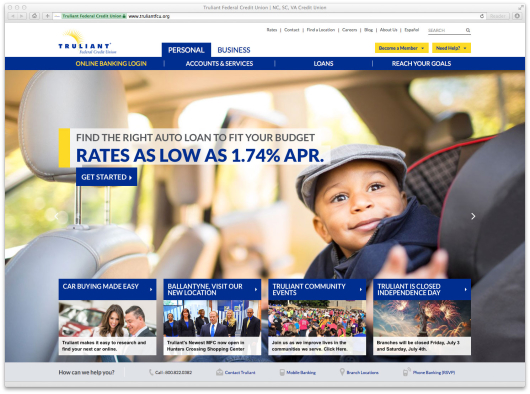The web page displayed is the business page of Truliant, prominently featuring the company's name in dark blue print on a white banner located at the top left corner. Adjacent to the text, a distinct yellow graphic resembling a ray of sunshine or a feather, emerges from the top of the letter 'L' in Truliant, extending gracefully to the left.

The page includes two main tabs: 'Personal' and 'Business,' with the 'Personal' tab currently open. At the forefront, highlighted by a blue background with gold lettering, is the 'Online Banking Login' section. Adjacent to it on the same blue strip are other navigation options such as 'Accounts and Services,' 'Loans,' and 'Reach Your Goals,' all displayed in white text.

The central visual element of the web page is an endearing photograph of a toddler, smiling slightly as he glances backward while seated in a car seat. His sparkling brown eyes are complemented by his light gray painter's cap and blue jacket. The car's interior features white leather seats, and the child's car seat is adorned with red piping and a brown and black checkered pattern.

Below the main image, additional clickable images lead to various sections of the website, including a category labeled 'Car Buying Made Easy,' accompanied by a relevant picture. Three similar sections are also visible, providing further options for exploration on the Truliant website.